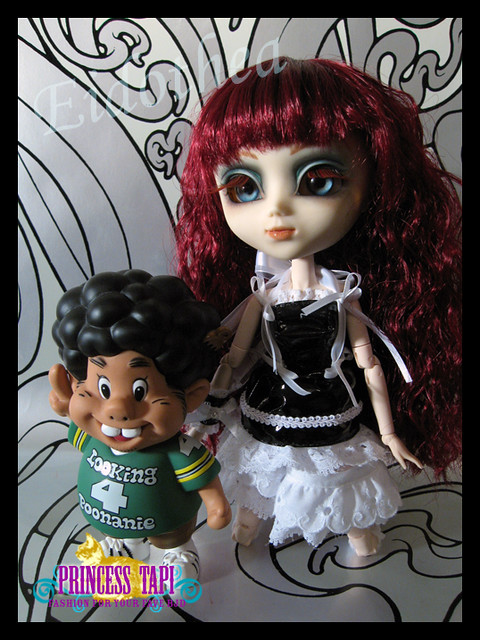In this image, there are two distinctive dolls positioned in front of a gray background featuring glowing swirls. The logo “Princess Tappi: Fashion for your...” is partially visible at the bottom. The doll on the left is a male, depicted with curly hair, large buck teeth, and dressed in a green football jersey with yellow stripes on the sleeves. The jersey has a racially insensitive slogan that reads, "looking for Poonani,” and the doll is also wearing athletic shoes. This portrayal seems to stereotype a Hispanic or Indian-American child, which can be viewed as borderline racist and tasteless.

The doll on the right resembles a Bratz doll and has a large head compared to its body. It features striking bright blue eyes with red eyelashes and matching reddish-purple curly hair. The doll is dressed in a gothic-style black gown adorned with white frills at the shoulders and a white slip underneath, reminiscent of characters from Tim Burton's "The Nightmare Before Christmas." The intricate costume and prominent facial details make it appear as a potential collectible from specialty stores like Hot Topic or Spencer Gifts.